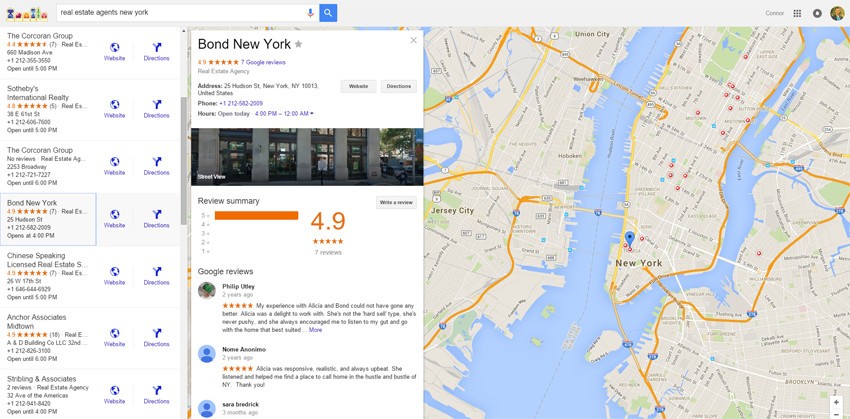This is a horizontal rectangular image, predominantly divided into two sections. 

On the right side of the image, there is a detailed map of New York. The map features the words "New York" prominently in black font, slightly below the actual midpoint. A notable blue teardrop with a black dot marks a specific location on the map, presumably the focus point. The map also highlights the rivers in blue and has an orange outline delineating certain areas.

To the left of the map, there is a vertical white section containing detailed information in black font. At the top, it reads "Bond, New York" followed by a star symbol. Below this, there are several orange-colored stars, though their exact content is partially obscured. Continuing downward, the text notes "seven Google reviews". Further down, address information is provided, followed by an exterior photograph of the hotel.

Beneath the photograph is the heading “Review Summary” followed by an orange number "4.9" towards the right of the center. This number is paired with stars that are nearly fully colored in orange, indicating a high rating close to five stars. Although the total number of reviews is difficult to discern, it is mentioned below the stars. On the far left side of the "Review Summary" section, there is a list displaying ratings from five to one, each associated with a horizontally filled orange bar, forming a bar graph representation.

Below this section, it states "Google reviews" and lists three specific reviews. All the way to the left, there is another list that appears to feature different hotels or groups, each with their respective contact information, though many details are hard to read. The name "Bond New York" stands out in this list, highlighted with a rectangle.